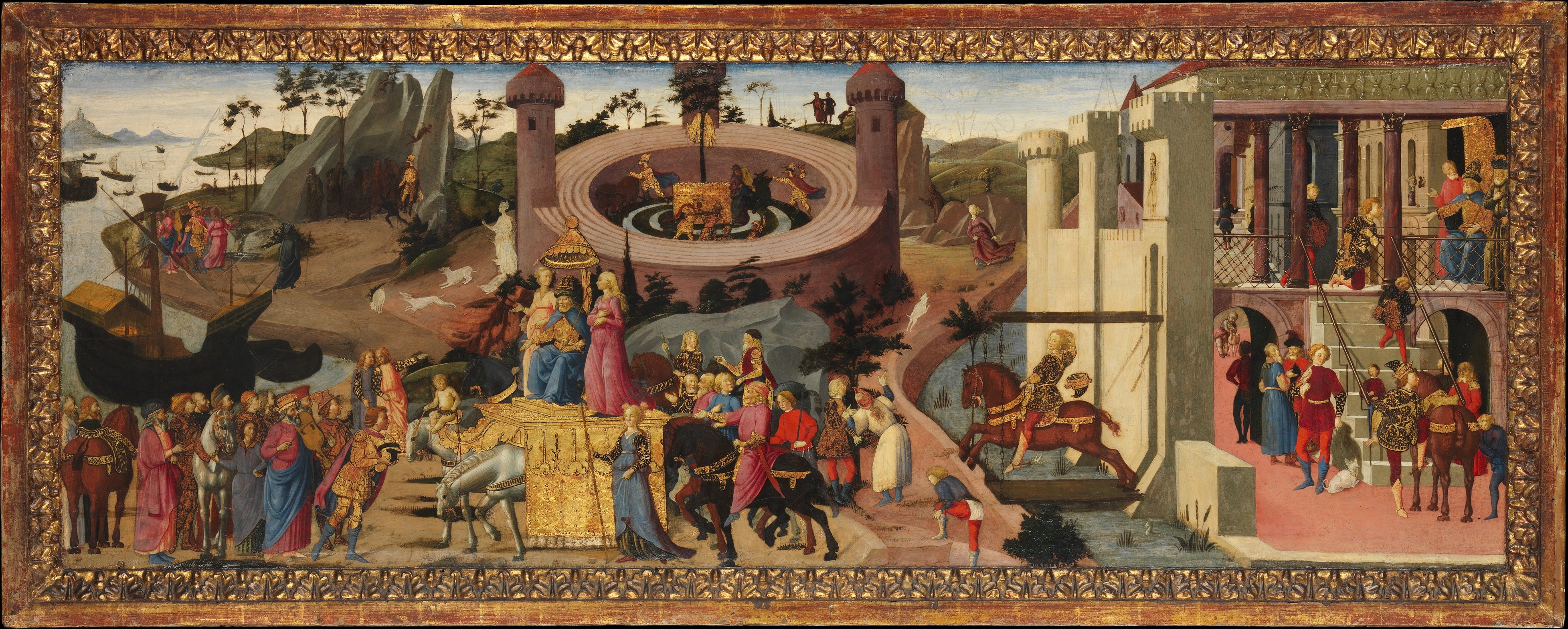This detailed panoramic painting, likely from the Renaissance period, captures an intricate medieval scene. The artwork is framed in a gold, bumpy-surfaced border, whose tactile quality adds to the overall classic aesthetic. At the center of the painting is a raised stage or pedestal, adorned in gold, where a figure resembling a king or an important personage sits on a throne. Flanked by two maidens, this central figure commands the attention of the surrounding crowds, who are all dressed in medieval attire.

The scene is bustling with activity and divided into segments. On the left, a large rock formation meets a landscape featuring a harbor or river with a black, old-style sailing ship reminiscent of a pilgrim's vessel. The right side showcases a meticulously detailed white castle with a drawbridge and fortifications. Inside, medieval-dressed individuals ascend white stairs to a second level. Another significant architectural element is a circular building with two watchtower-like structures, possibly a coliseum or a royal venue, positioned symmetrically behind the central stage.

Horses play a significant role in the composition, with one horse positioned under the pedestal and another drawing a vehicle carrying the central figure. A third horse crosses from the castle foreground via a drawbridge over a small moat. The painting is rich with reds and blues, drawing the viewer's eye to specific areas and figures. Overall, this captivating work presents a dynamic tableau of medieval life, accentuated by the various architectural and natural elements that frame the bustling human activity.